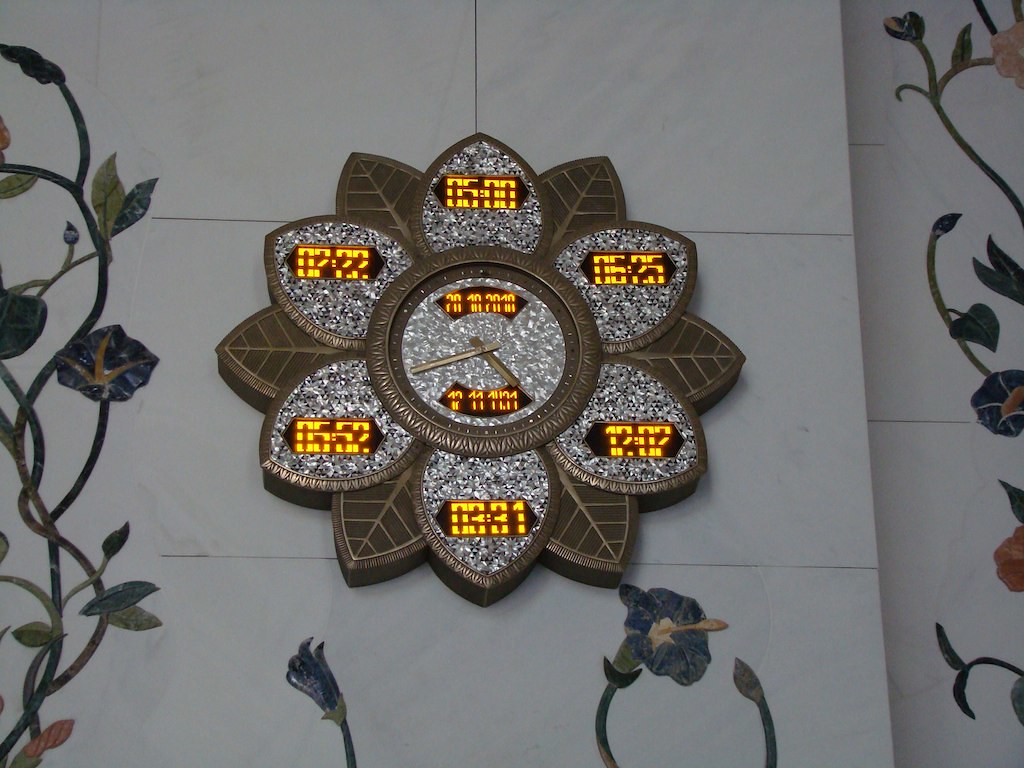The photograph depicts a highly intricate, possibly AI-generated digital clock designed in the shape of a flower, positioned on a dark grey tiled wall. The central circular section of the clock is surrounded by glittery silver petals interspersed with darker brown, copperish petals with leaf veining. The central face of the clock has a mothballed grey appearance and is adorned with light metallic clock hands. These hands appear to point to different times on various occasions: 5:00, 7.22, 5.52, 3.31, 12.02, and 6.25. The clock features dark panels at both the top and bottom of its middle section, displaying blurred yellow fluorescent digital numbers, indicating times possibly programmed for multiple time zones.

Surrounding the clock are additional digital screens embedded within the floral design, showing similar yellow lighting. The decor incorporates a floral trellis design with blue and red flowers intertwined with green tendrils, enhancing the organic aesthetic against the tiled wall. The background tiles feature lines and leafy patterns, adding to the overall detailed and ornamental look of the image.